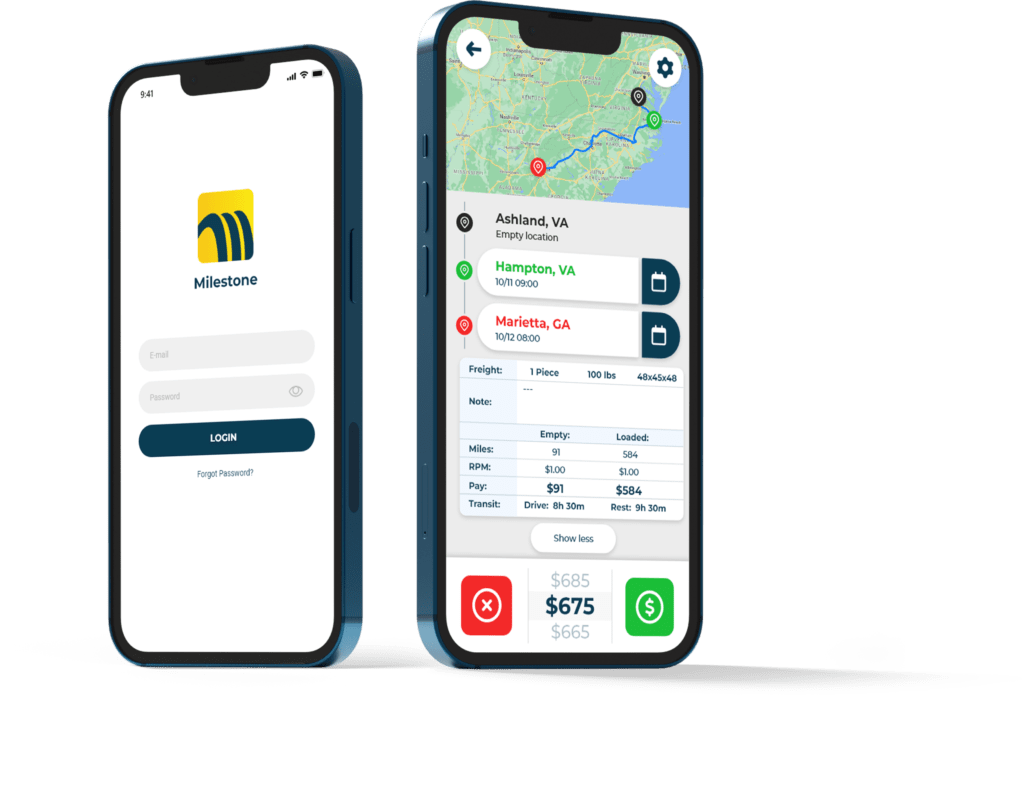In this image, we are presented with a detailed screenshot displaying two smartphones, each angled slightly away from the viewer. The phone on the left is slightly turned to the left, while the phone on the right is angled to the right. Both phones are encased in black covers, or they might be black in color.

The screens on both devices are illuminated. On the left phone, set against a white background, the status bar at the top indicates the time as 9:41 AM, full reception, Wi-Fi connectivity, and a fully charged battery. Prominently displayed below is a yellow square containing black icons, labeled "milestone." Further down, there is a black text box with white text prompting the user to log in, accompanied by an option to recover a forgotten password.

The right phone's screen features a map occupying the top third, showcasing a green landscape with a blue directional line and a red circle marking the destination. Text beneath the map provides travel details: "Ashland, Virginia to Hampton, Virginia, 10/11 at 9 o'clock," followed by, "Marietta, Georgia, 10/12 at 8 o'clock." This structured display offers a comprehensive view of the phones' screens, emphasizing both the functional and navigational aspects of their current usage.